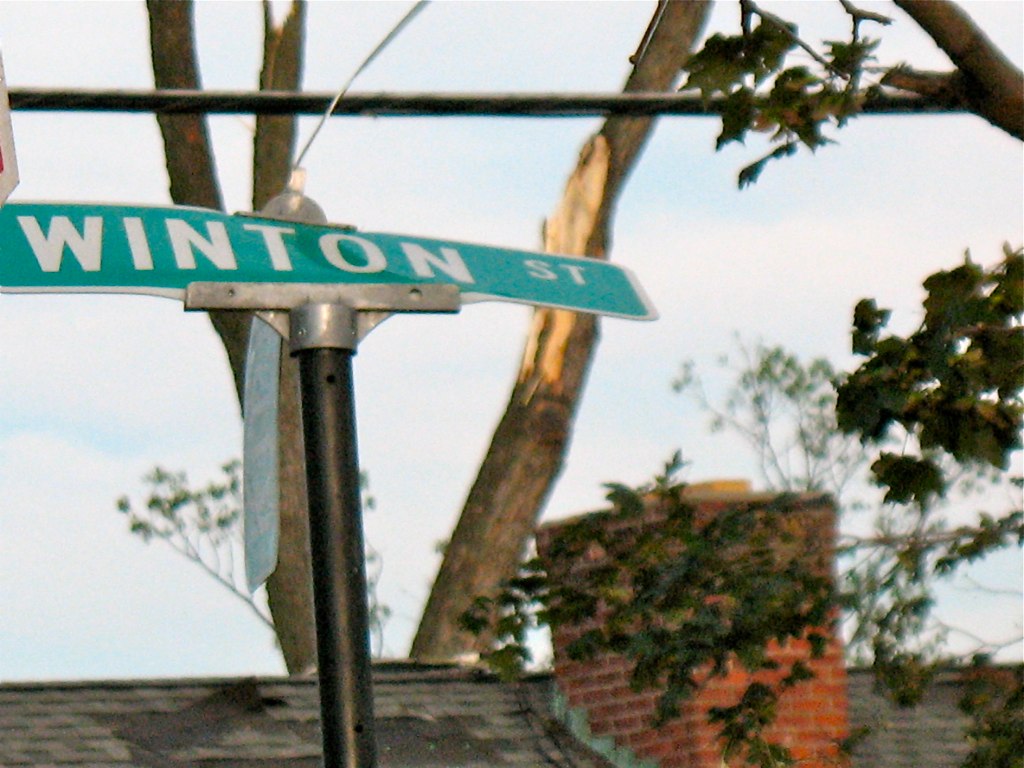This rectangular, landscape-oriented outdoor photo captures a high vantage point view of a green street sign that reads "Winton." The sign, with rounded corners and a white edge, is noticeably bent backward at the top of the pole it is mounted on. The background reveals a serene, pale blue sky adorned with wispy clouds. The sun's reflection graces the leaves of a tree, whose branches extend behind the roof of a house featuring a brick chimney. In the distance, more trees are visible, characterized by tall, slender branches and clusters of leaves. Another tree and possibly another pole intersect near the top of the image, contributing to the layered composition of urban and natural elements.